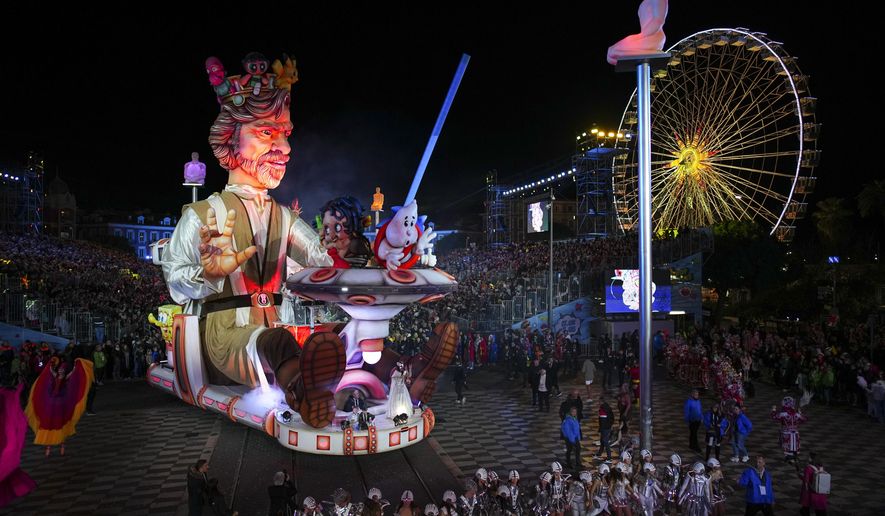This nighttime photograph captures a vibrant scene at a grand festival or amusement park, composed in a horizontal rectangular format. Dominating the center of the image is an impressive multi-story parade float, three to four stories high, which features a statue of a Star Wars character holding a lightsaber and raising his hands. The float, which reflects off a paved surface, is surrounded by a large crowd of spectators. Many attendees are dressed in Star Wars costumes and helmets.

Behind this central figure, slightly off-center to the left, is another elaborate float depicting a king with brown hair and a crown, seated at a table. In the far background, a gigantic, brightly lit Ferris wheel glows against the black night sky. Adjacent to the Ferris wheel, additional amusement park rides and metal scaffolding enhance the festive atmosphere. The entire scene is teeming with people both in the foreground and packed stands, all absorbed in the spectacle of the parade.